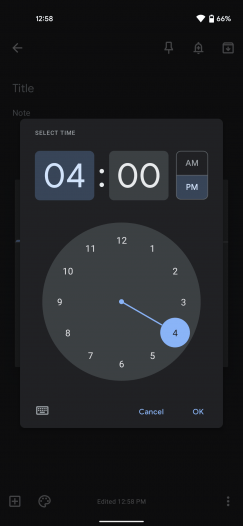Here's the cleaned-up, detailed caption for the image:

The screenshot of the phone displays an interface with a black background. At the top, in white text, the time is shown as 12:58. On the right side of the top bar, icons for Wi-Fi and battery are visible, with the battery percentage indicated as 66%. Below this bar, several light black icons, including an arrow for going back and a few other symbols, are positioned on the right.

The primary focus of the screen is a clock interface dominating the center. At the top of this interface, two squares indicate the current time settings: "04," followed by two white dots, and "00," with buttons for AM and PM beside them. These elements are rendered in different shades of black with white text.

Below this, there is a large circular clock face displaying numbers from 1 to 12 around its perimeter. A blue line extends from the center of the clock to a blue circle around the number 4, marking the selected time. Towards the bottom of the screen, an icon is present on the left, while "Cancel" and "OK" buttons are placed on the bottom right in a purplish color.

Finally, at the very bottom, additional icons are arranged, including three dots on the right and a small horizontal line at the very bottom, all depicted in black.